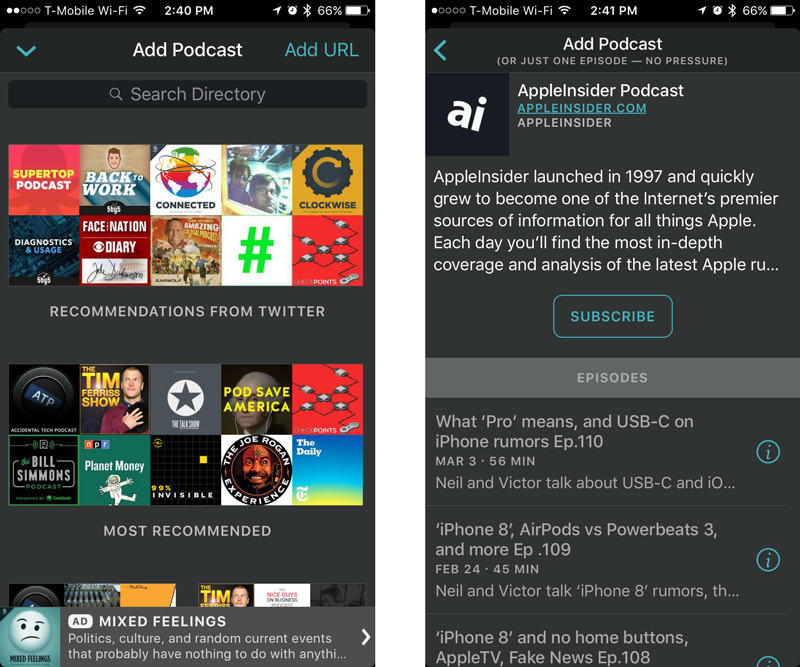This image features two screenshots from a smartphone, both showcasing different stages related to podcast discovery and subscription. 

In the first screenshot, the user is utilizing the search function on their device to locate a specific podcast of interest. Prominently displayed across the top is a search bar, indicating active user input. Below the search bar, there are several small squares highlighting recommended podcasts, potentially curated based on user interests. These recommendations are further split into two sections: "Recommendations from Twitter" at the top, and "Most Recommended" positioned further down.

The second screenshot appears to show the result of the user's search selection, focusing on the "Apple Insider Podcast." This podcast is produced by appleinsider.com, and a brief description beneath the title reads, "Apple Insider launched in 1987 and quickly grew to become one of the Internet's premier sources of information for all things Apple." Below this description, there is a conspicuous grey button with blue text reading "SUBSCRIBE," inviting users to subscribe to the podcast if they find it appealing. The podcast's icon features the lowercase letters "ai," angled slightly sideways towards the top right. Underneath the podcast's icon and description, there is a list of episodes available from the podcast, ready for listeners to explore.